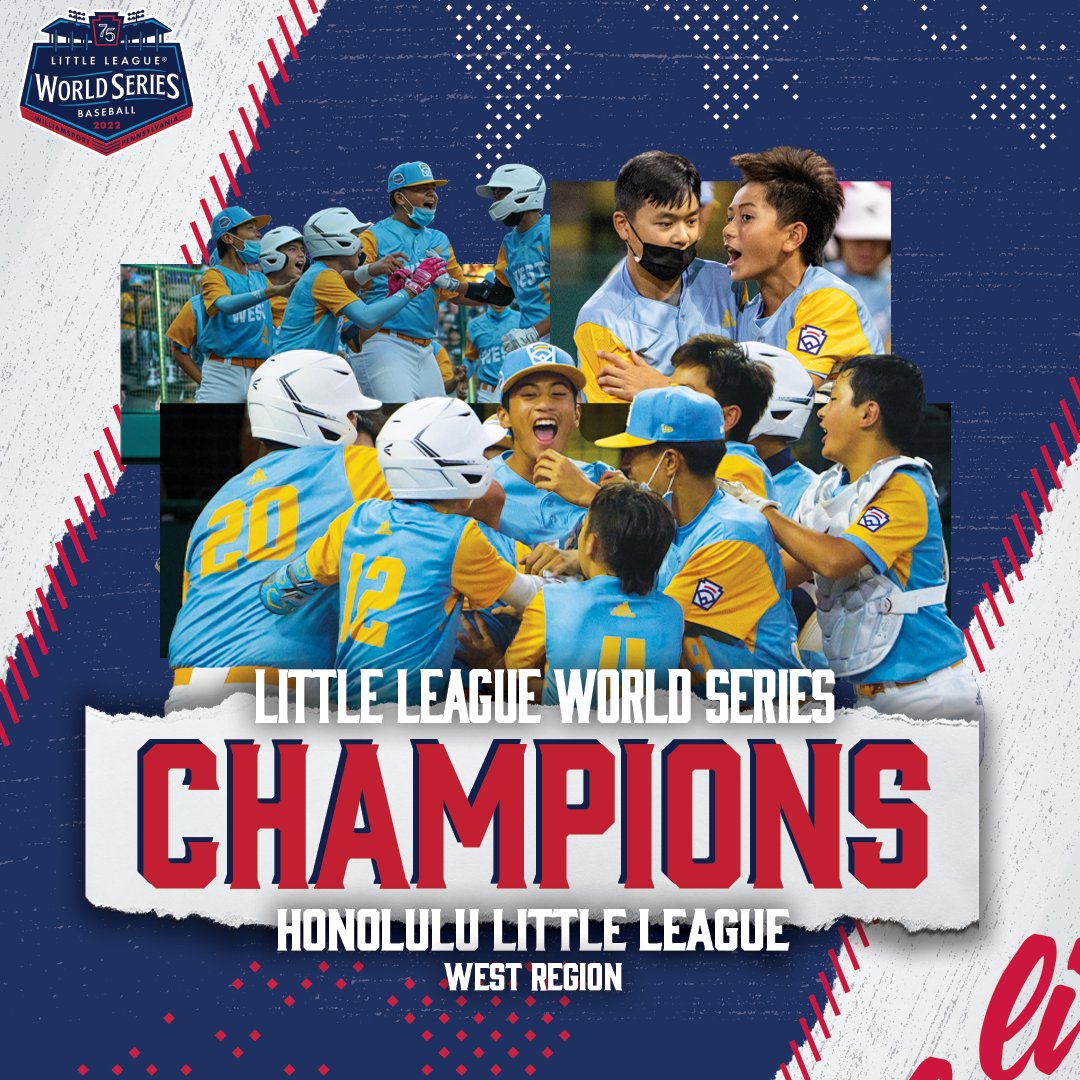The advertisement for the 2022 Little League World Series champions, Honolulu Little League from the West Region, prominently features the team in celebration. The main image shows the young athletes huddled together, adorned in light blue jerseys with yellow sleeves and numbers, and blue hats with yellow bills. Central to the scene, a smiling player catches the joyful attention of his teammates, possibly the winning pitcher. Surrounding the central image, smaller action shots capture additional moments of victory, showing players in helmets and face masks celebrating passionately. At the top left, the poster includes the Little League World Series Baseball logo and the number 75, signifying the 75th anniversary of the event. The backdrop melds a patriotic red, white, and blue color scheme with stitching reminiscent of a baseball, enhancing the celebratory and authentic feel of the advertisement.